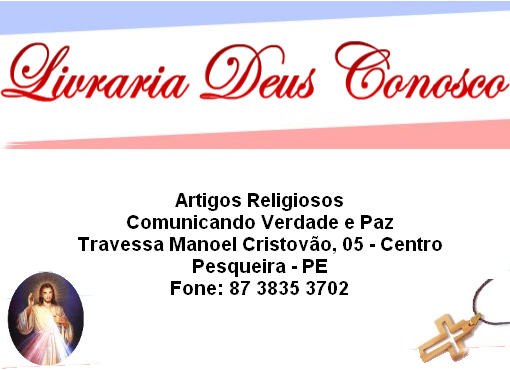This image is a business card or advertisement likely from a church in another country, written in what appears to be Portuguese. Across the top in red cursive font, it reads "LIVRARIA DEUS CONOSCO." Beneath that, in black sans serif font, it states "Artigos Religiosos," followed by "Comunicado Verdad e Paz," which translates to "Truth and Peace Communication." Further down, it provides an address: "Travesa Manuel Cristovão, 05 Centro," indicating "Pesqueira PE" along with a contact number: "87-3835-3702." The bottom corners of the card feature religious imagery, with a cross in the bottom right corner and an image of Jesus in the bottom left corner. The card seems to be promoting religious items and services.